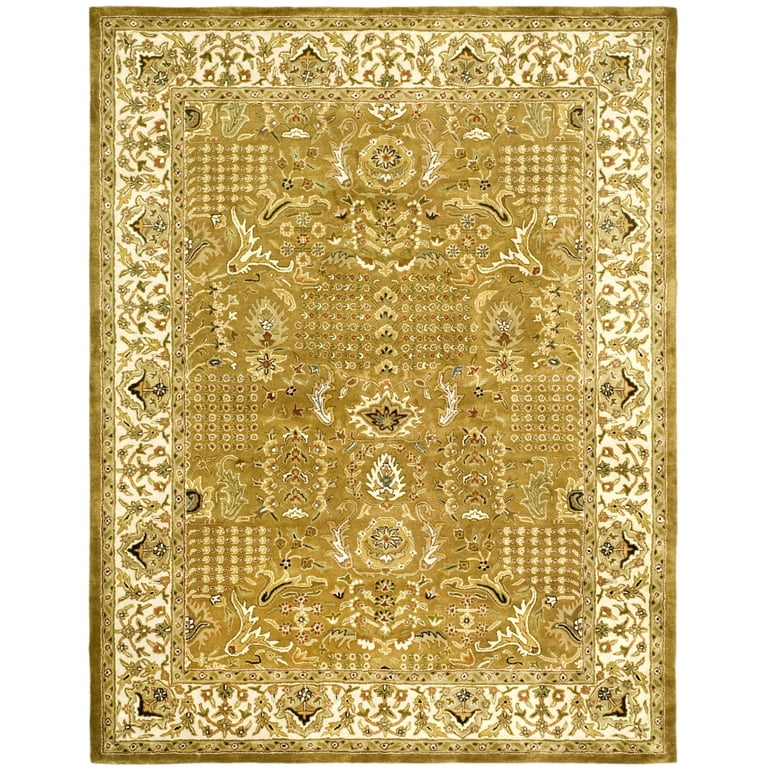A detailed description of the intricate rectangular carpet rug emphasizes the prevalent elements shared in the provided captions. The rug features a light gold border that transitions from light to dark hues. Just inside this border is a thin lining with a lighter gold color, adorned with small black dots and delicate gold weaving.

Moving inward, there's a white background rectangle, intricately lined with etchings resembling brown houses with purple arched roofs, forming a continuous pattern across the top, sides, and bottom. The central section comprises another rectangle containing several segments with light gold-colored dots arranged in a grid formation. At the center of this section is a distinct black star-like shape with an extended top, surrounded by white points. 

Additionally, a particular area displays a white emblem resembling a Christmas tree. Despite the presence of some facial and flag-like designs noted towards the center, the overall aesthetic of the rug is dominantly gold and beige, with variations that include beige, brown, black, and subtle blue accents forming intricate patterns reminiscent of leafy or fluffy shapes and lines. This creates a rich yet subtle visual complexity suitable for beige color enthusiasts. From afar, the rug may appear to have a slightly dirty white or light beige tint due to its intricate design.